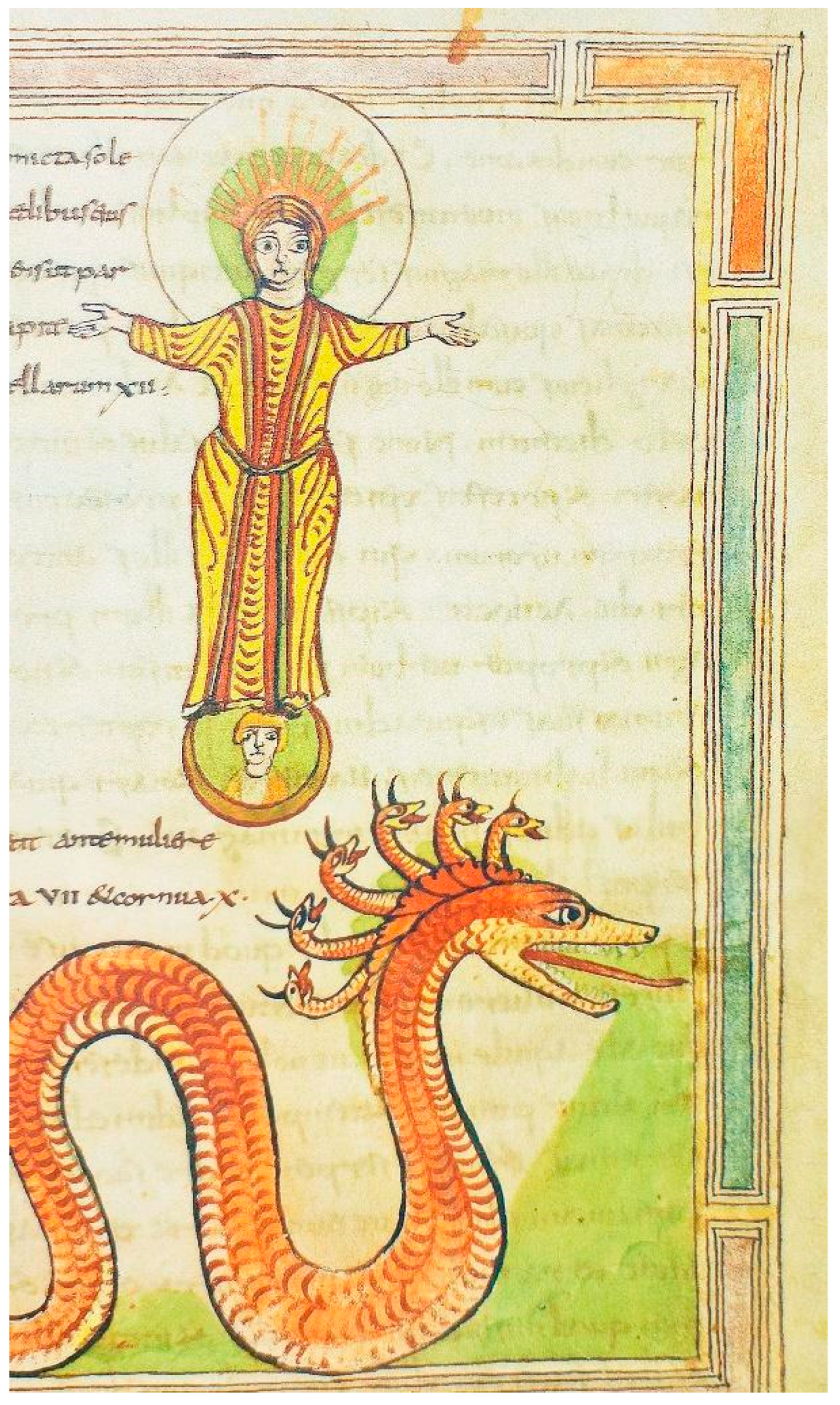This is a rectangular print that appears to depict a religious figure at its center. The figure, a white person, is dressed in a yellow robe with orangish-red accents and has arms outstretched. The figure wears an orange crown adorned with long spikes, which is surrounded by a green aura, suggesting a halo effect. The background includes some writing in an unknown language, with text present both in the upper left-hand corner and below the central image.

The figure stands atop a semicircular structure, within which a smaller figure with yellow hair is depicted, likely signifying a mirror or reflection. The second figure does not resemble the central figure, adding a layer of mystique to the composition.

At the bottom of the print is a large, snake-like dragon, predominantly orange, with its mouth open and tongue extended. This snake has six additional dragon heads protruding from the back of its main head, all similarly open-mouthed with extended tongues. Lime green accents are scattered throughout the image.

The entire scene is framed by a multicolored border with sections of lavender, orange, aqua, beige, and yellow, though it appears faded with age, lending a timeless quality to the artwork.